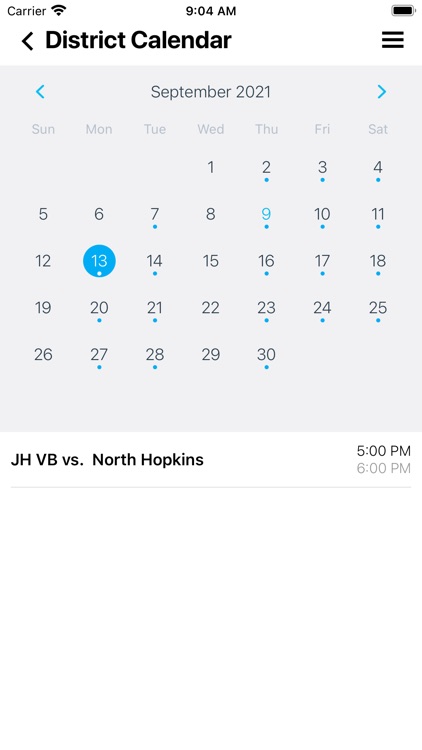A detailed screenshot of a mobile phone displaying a calendar for September 2021. In the top left corner, the word "Carrier" indicates a strong signal alongside the full battery icon. The current time is 9:04 a.m. The calendar highlights September 9th, a Thursday, in blue, suggesting that this screenshot was taken on that day. Another notable date, September 13th, is encircled in blue, indicating an important event. The area below the calendar provides further context with a reminder: "JHBB vs North Hopkins at 5 p.m. to 6 p.m.," suggesting that the 13th is bookmarked for a sports match.